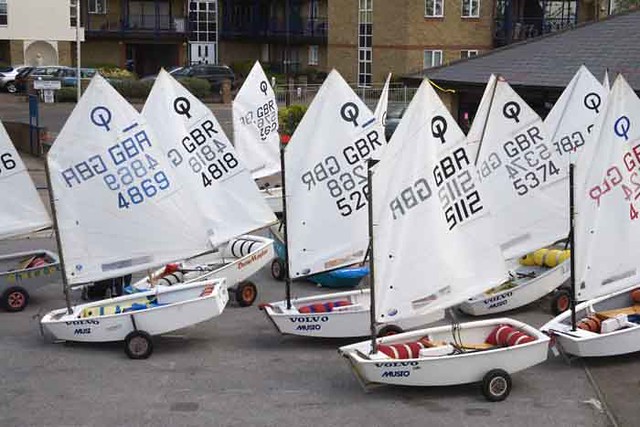In this outdoor urban scene, several small white sailboats are lined up on gray, slightly aged and splotched pavement, each secured on wheeled tow trailers. These boats, which resemble miniature sailboats with their white bodies and single white sails, each bear distinct identification numbers such as GBA 5112, GBR 5374, and GBR 4869, suggesting they might be prepared for a race or competition. Red and white striped pillows are seen inside each boat. The backdrop features a row of connected older buildings, including brown brick structures with white-trimmed windows, a darker building, and a cream-colored one. Parked cars can also be seen amidst this urban setting.